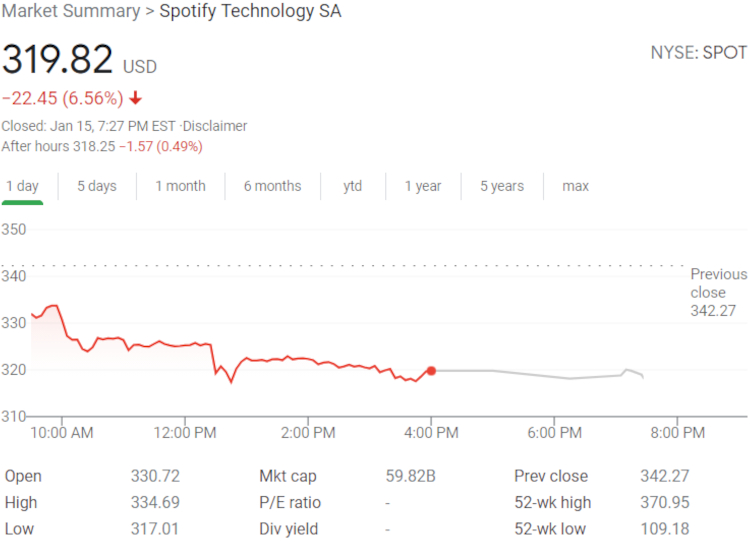This image displays a stock market summary for Spotify Technology S.A. (NYSE: SPOT). Key details are as follows: 

- **Stock Price:** $319.82 USD per share, a decrease of $22.45 or 6.56%.
- **After-Hours Trading:** The price dropped further to $318.25, a decrease of $1.57 or 0.49%.
- **Market Closure:** January 15th at 7:27 PM Eastern.
- **Price Chart Timeline:** The chart illustrates the stock's performance over a single day, from 8 AM to 8 PM.
- **Opening Price:** $330.72
- **Daily High:** $334.69
- **Daily Low:** $317.01
- **Market Capitalization:** $59.82 billion
- **Previous Closing Price:** $342.27
- **52-Week High:** $370.95
- **52-Week Low:** $109.18

The chart reveals a general downward trend throughout the trading day, underscoring a significant decline in the stock price. The dramatic difference between the 52-week high and low points out the volatile nature of the stock, indicating potential for both substantial gains and losses for investors.